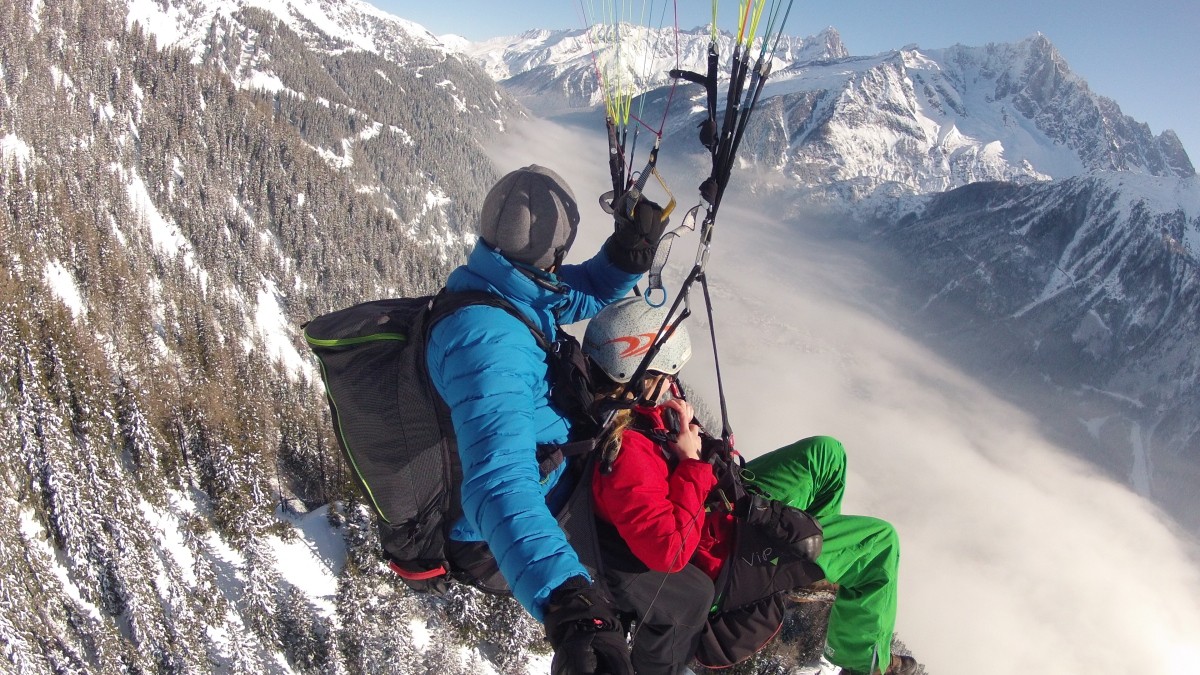This breathtaking photograph captures two people paragliding high above a stunning mountainous landscape. The person on the left, who appears to be a man, is wearing a puffy blue jacket, dark pants, black gloves, and a gray helmet. He has a long black backpack on his back and is holding onto the paragliding gear with cords extending out of the frame above them. In front of him, securely strapped in, is a woman wearing a vibrant red jacket, green pants, and a distinctive gray helmet with red arrows. They both are completely suspended in the air, seemingly gliding effortlessly over the majestic snow-covered mountains and dense forests below. To their right, a deep valley is shrouded in a dense, dark gray mist, contrasting with the brilliant blue, cloudless sky above. The perspective of the shot suggests the man might be using a selfie stick to capture this exhilarating experience from a dynamic angle, further accentuating the dramatic scenery and the thrill of paragliding.